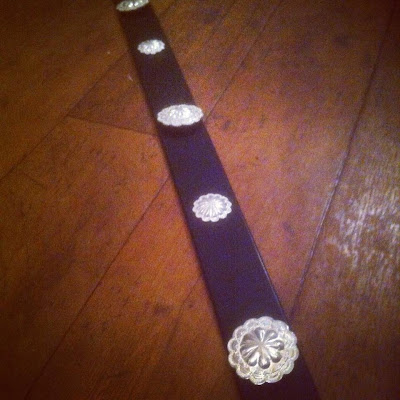This is a detailed photograph of a black belt, about half an inch wide, adorned with five silver buckles. The belt lies flat on a wooden floor, which is brown with varying shades and textures, suggesting it might be an old and well-worn hardwood surface that has been recently polished, giving it a bit of shine. The silver buckles feature a flower design in the center with scalloped edges, resembling sand dollars. The belt's position is slightly diagonal, somewhat off-center in the image. The photograph is small, approximately two by two inches, capturing only the belt and the floor with no additional objects, people, animals, text, or identifying information. The lighting is fairly bright, illuminating the belt and enhancing the details, although the overall image quality could be better.